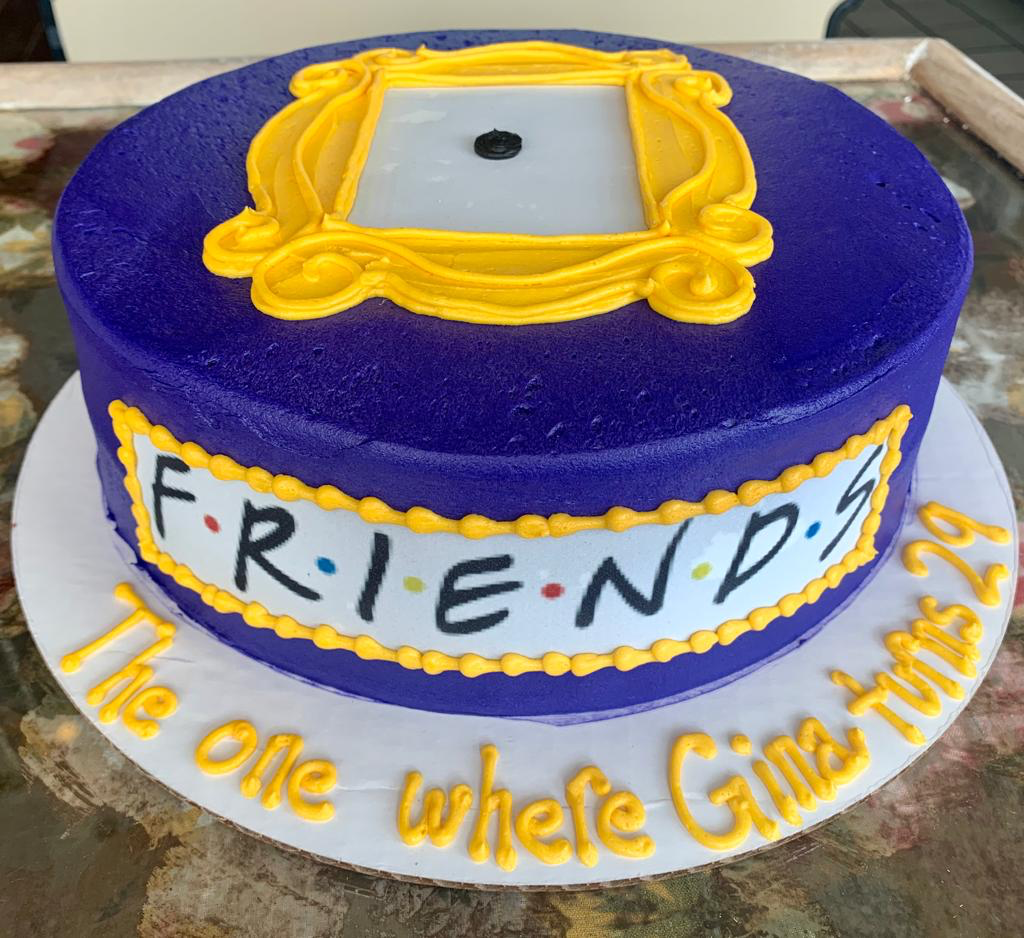This photograph showcases a carefully crafted, circular cake inspired by the Friends TV show. The cake's main body is coated in dark royal blue fondant icing. Prominently displayed on the side of the cake is the Friends logo, meticulously rendered in black lettering on a white background, adorned with red, blue, and yellow dots between the letters. On top of the cake is a bright yellow icing depiction of the iconic picture frame from the peephole on the apartment door from the show, complete with a small black dot representing the peephole center. The cake is placed on a cardboard base, which sits atop a sophisticated gray and brown marble tray or tabletop. In front of the cake, written in yellow icing, are the words "The one where Gina turns 29," embracing the show's episode-naming style. This edible art captures the essence of the Friends theme, making it a perfect homage for a fan's 29th birthday celebration.